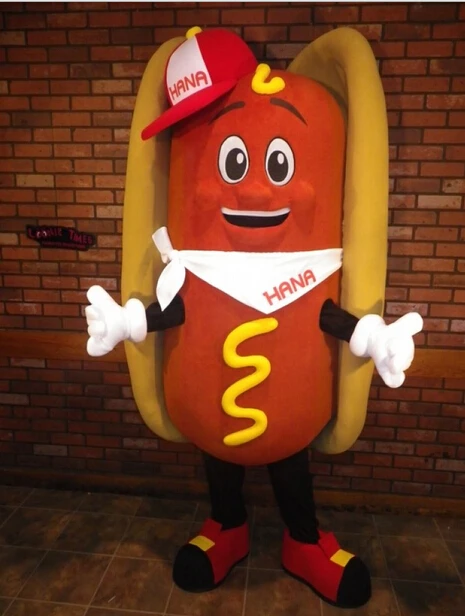In this colorful, portrait-oriented photograph, an adult-sized mascot costume of a smiling anthropomorphized hot dog stands against a red brick wall, with brown-tiled flooring beneath. The bright red hot dog is sandwiched between two bun halves of a bread color, complete with a swirl of yellow mustard starting at the forehead, continuing under a white bandana, and trailing down the body. The hot dog character sports a red and white baseball cap, tilted jauntily to the left, and marked with the name "Hannah" spelled out as H-A-N-N-A in red lettering. Matching the cap, the white bandana around the neck also carries the name "Hannah." The character features large cartoonish white gloves, black sleeves, black leggings, and red and black sneakers with a stylized gold buckle. The hot dog smiles warmly at the viewer, adding a fun and inviting touch to the playful scene.